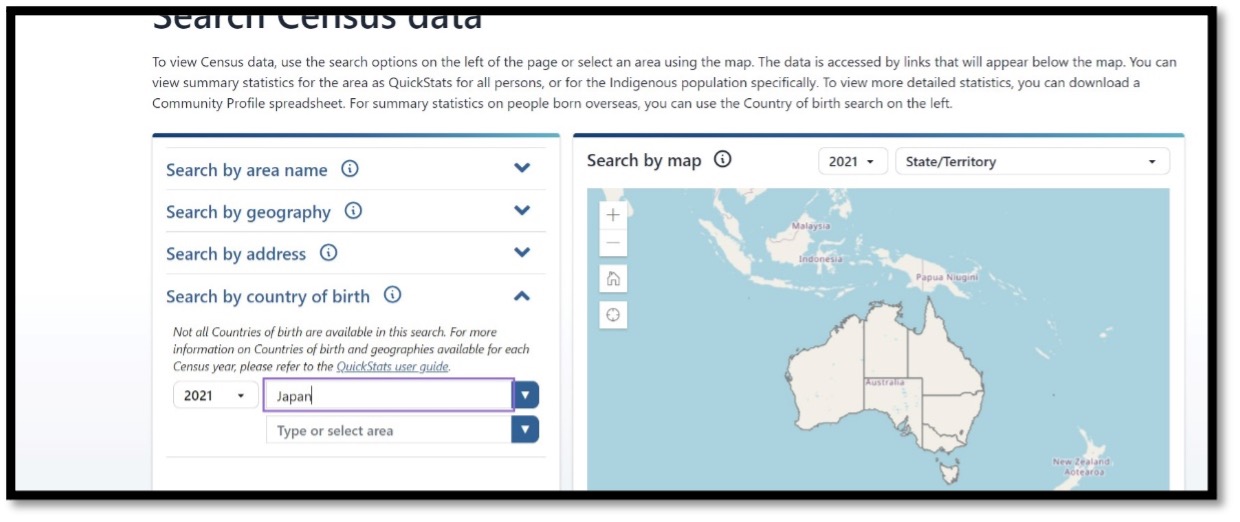The image displays a portion of a webpage with a white background and black text, neatly framed by black lines. The header reads "Search Census Data." Below the header, there are instructions on how to access various census data. It notes that users can view census information by selecting options on the left of the page or by clicking on an area within a map. 

The instructions indicate that links to specific data will appear beneath the map, offering summary statistics through quick stats. These statistics can include data for all residents or specific demographic groups, such as the Indigenous population. For accessing more detailed statistics, users are directed to download a community profile spreadsheet.

The search options provided include "Search by Name," "Search by Geography," "Search by Address," and "Search by Country of Birth." There is an additional note stating that not all countries of birth will be available in the search, and for details on available countries and geographies for each census year, users should refer to the "Quick Stats User Guide."

At the bottom of the screenshot, there is a text entry for "2021 Japan," accompanied by a map of Japan, although the map is not highlighted, suggesting that Japan might not be available in the immediate search results and may require consultation of the Quick Stats User Guide for more information.